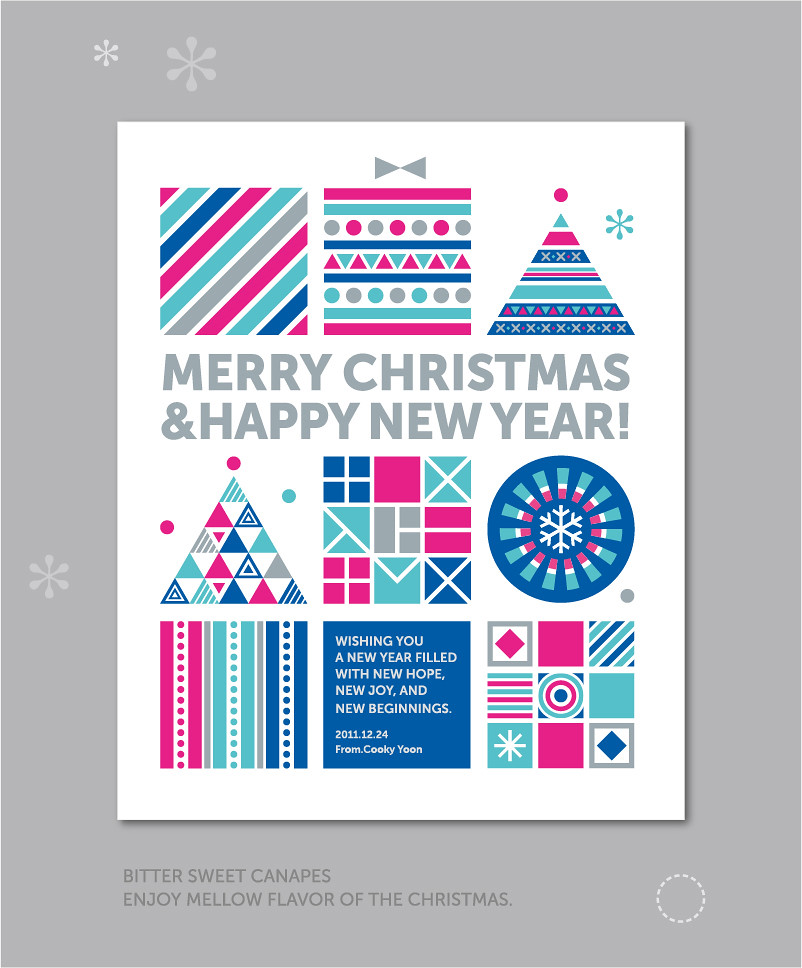This image depicts a festive Christmas card with a gray background and a light gray border adorned with three rounded snowflakes— two in the top left corner and one on the left side. At the bottom of the border, in dark gray text, it ambiguously reads, "bittersweet canapes enjoy mellow flavor of the Christmas."

The centerpiece is a white rectangle filled with geometric illustrations of Christmas presents and trees, rendered in shades of red, pink, blue, light blue, green, and gray. These shapes include triangles (some representing Christmas trees topped with a red dot as an abstract star), squares, and circles, arranged in a playful, vibrant collage. In the center of this white space, the greeting "MERRY CHRISTMAS AND HAPPY NEW YEAR" is displayed prominently in gray uppercase letters. Below this, another message states, "Wishing you a new year filled with new hope, new joy, and new beginnings," alongside the date "2011-12-24."

The visual and textual elements combine to create a cheerful and modern holiday greeting card.